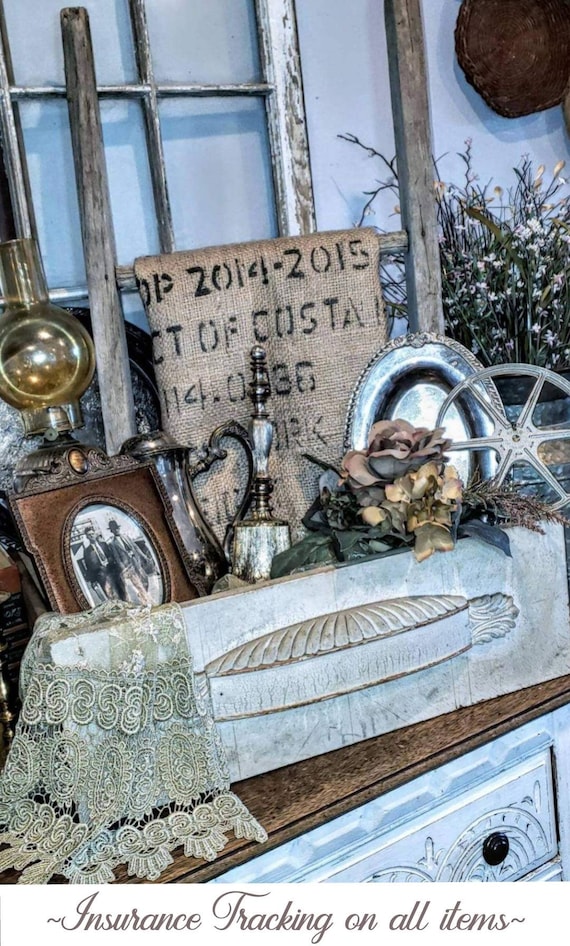The image shows a curated assortment of vintage items possibly for an insurance inventory, laid out on a pristine white chest of drawers with a brown wooden top, positioned against a white wall. A collection of intriguing objects are meticulously arranged, including a large lace cloth with delicate embroidery, a silver serving tray, and an old-fashioned gas lamp. An embossed wall plaque, resembling a cake pan or a wheel, hangs above the dresser. A striking old-fashioned western photograph in a brown leather frame, an oil lamp, and a burlap sack marked with the years “2014-2015” and the word “Costa” add to the nostalgic ambiance. A rustic atmosphere is further evoked by the barn wood windows and display racks in the background, alongside a large wash tub cradling a vibrant plant with white flowers. There's a sign at the bottom of the image that reads "insurance tracking on all items," suggesting that these items have been carefully documented for insurance purposes.